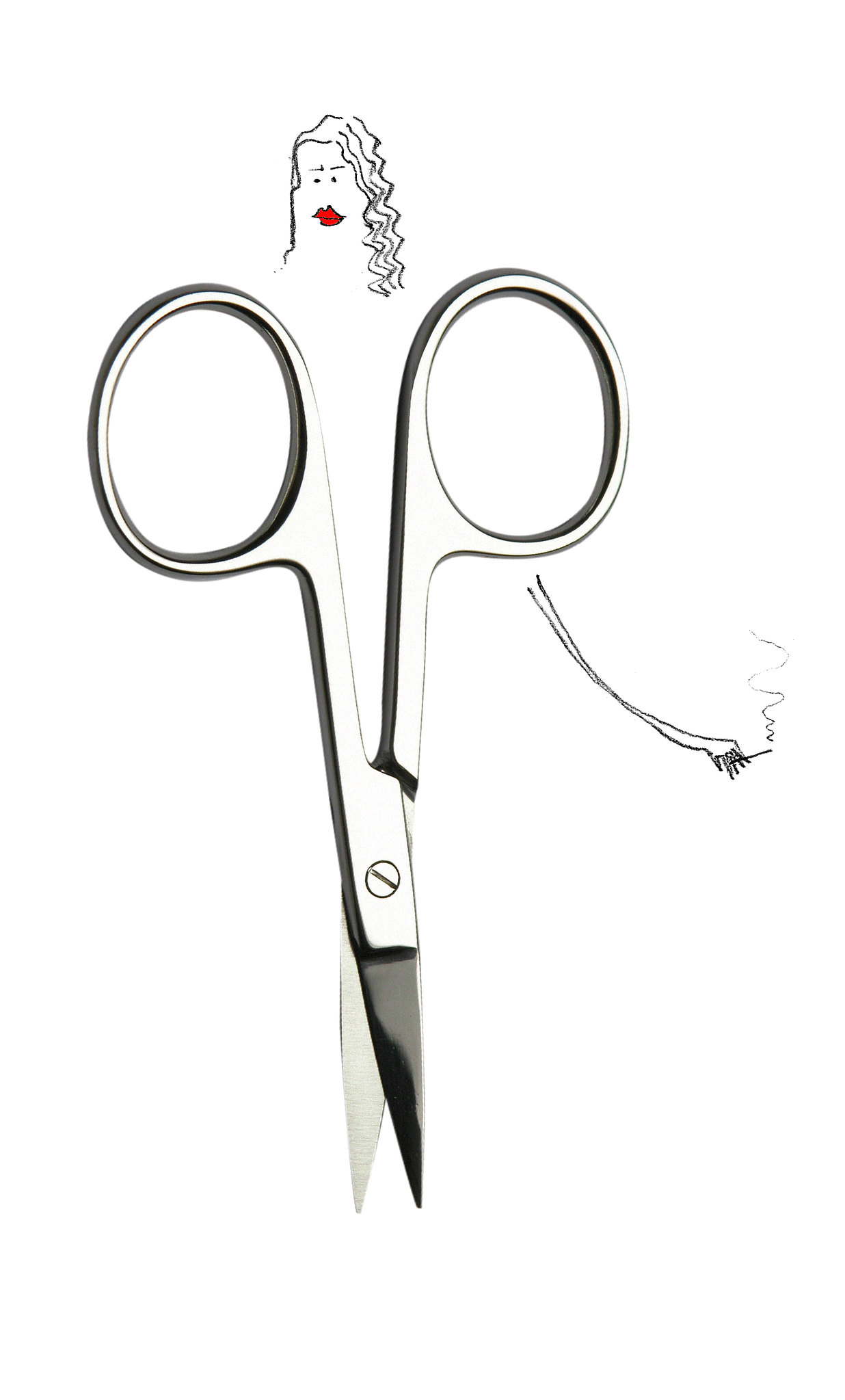This illustration features a pair of small, vertical, stainless-steel scissors, positioned upside down against a white background. The handles of the scissors extend upwards, forming the body of a woman’s figure. At the top, replacing the traditional scissor handle, there is a detailed ink drawing of a woman's head. She has black hair flowing predominantly to the right, dark eyebrows, expressive black eyes, and striking red lips. A slender, thin arm extends from the right side below the head, delicately holding a lit cigarette with a small wisp of smoke curling upward. The screw joining the two blades of the scissors at the center is clearly visible, and the blades taper down to fine, needle nose tips, giving a darker silver hue towards the bottom. The entirety of the illustration suggests the scissors collectively form the woman’s torso and legs, blending practical object with whimsical, artistic elements.